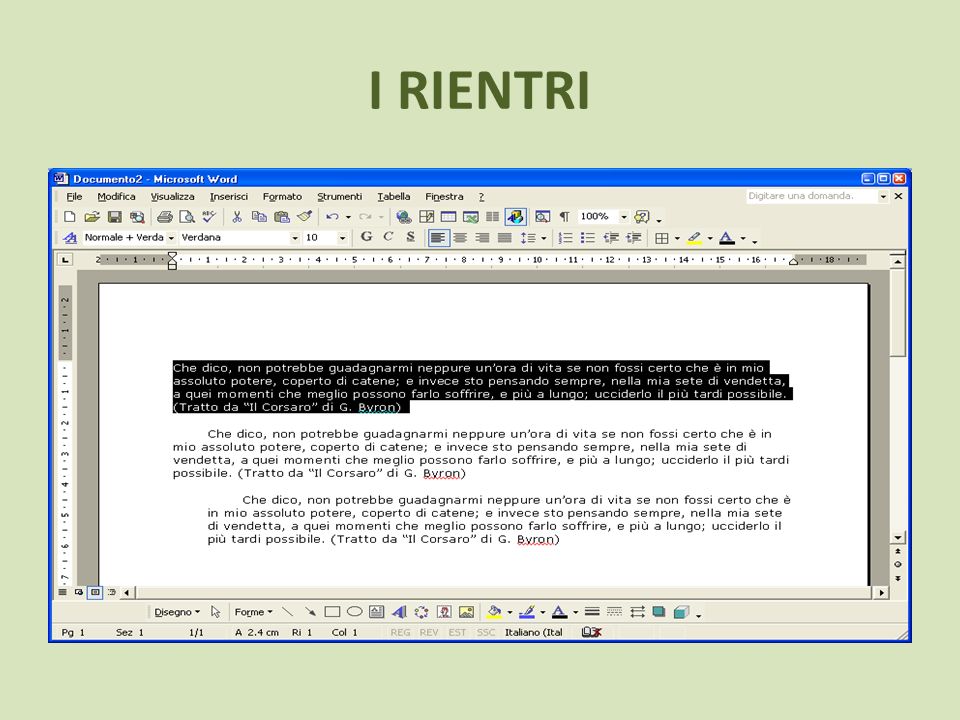The image is a detailed screenshot of a Microsoft Word document prominently displayed on a computer screen. The overall background of the image is a horizontal rectangle with a grayish solid color. Centered in the image is a screenshot set against a lime green backdrop. The title at the top of the screenshot reads "I R-I-E-N-T-R-I" in dark green letters, suggesting the document might be in Italian. Below the title, the screen displays a Word document named "Documento 2," consistent with Italian nomenclature. The Word interface menus are in Italian, with options like "File," "Modifica," "Visualiza," "Inserciza," and "Formato." 

The document itself contains three paragraphs of text. The top four rows of text are highlighted in black with white lettering, while the remaining portions of the document have standard black text against a white background. Notably, the first two paragraphs appear to begin with the word "Cedico," though they differ in precise wording. The third paragraph is also not highlighted but maintains the same formatting style. Various colors, including light green, dark green, blue, white, black, yellow, turquoise, and red, are seen throughout the image interface, adding a vivid contrast to the overall depiction.